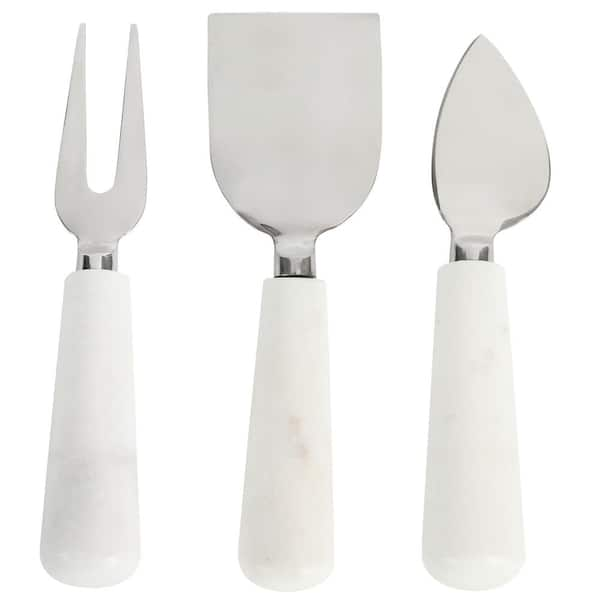This image features a trio of elegant, silver-topped hors d'oeuvre serving utensils, set against a pristine white background. Each utensil possesses a short, chunky handle that tapers from a narrow top to a wide, rounded bottom, all in a matching white color. To the left is a broad, two-pronged fork, ideal for spearing olives or slices of salami. In the center lies a solid, flat-headed spatula, perfect for cutting softer cheeses like brie. The utensil on the right is a leaf-shaped cutter with a dull point, designed for scooping and spreading items such as soft cheeses onto crackers. Despite their sophisticated purpose, the utensils appear notably dull and dimly lit in the photo.